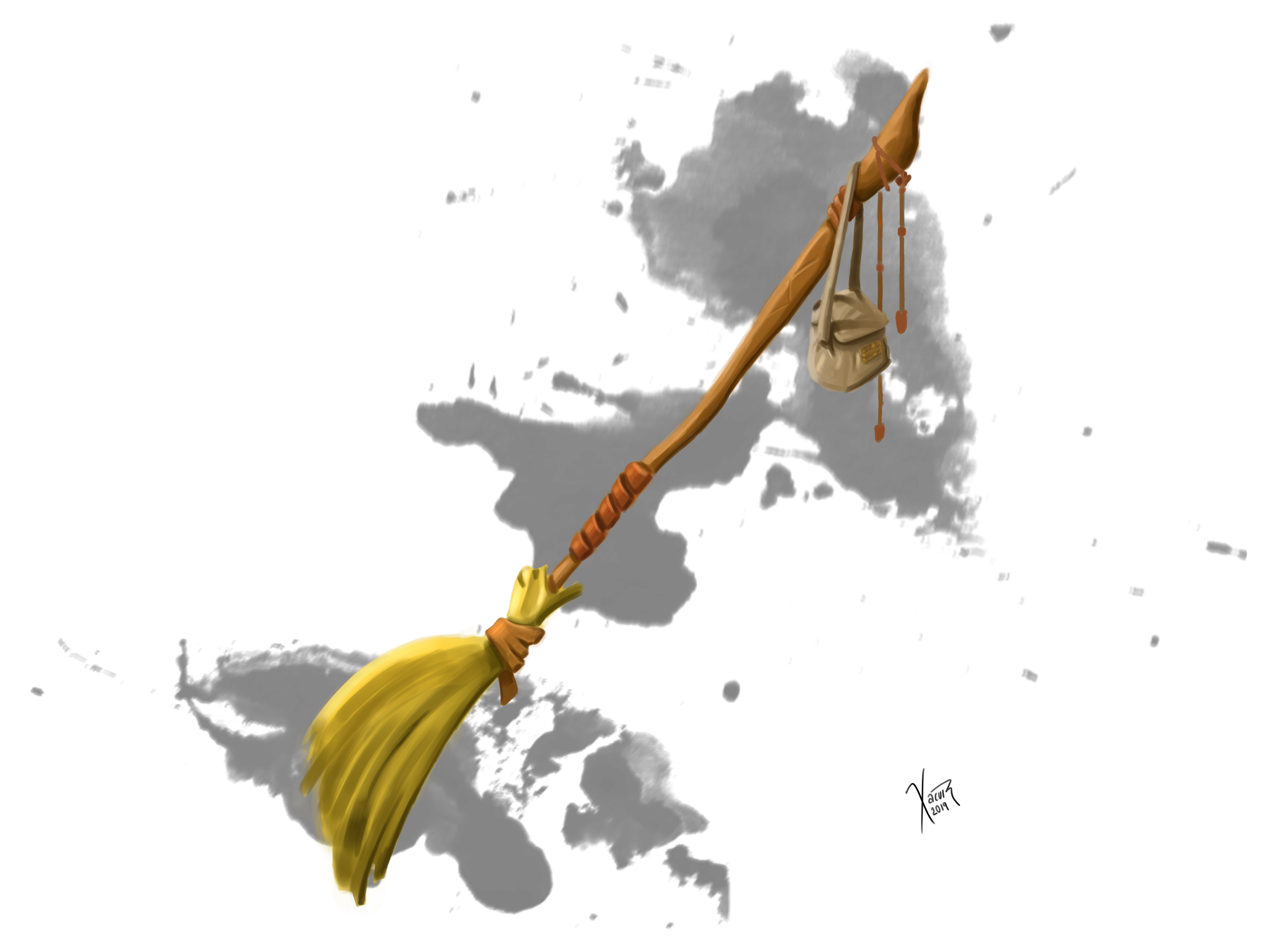This detailed artwork features an animated drawing of a broom diagonally aligned from the lower left to the upper right of a white background. The bristles, which are bright yellow, are situated in the lower left corner, transitioning to a wooden brown handle that slightly curves as it stretches toward the upper right corner. The broom handle is adorned with three horizontal bands of darker brown material, resembling leather, and exemplifying a rustic, natural appearance. Dangling from the top of the handle is a small, grayish-tan handbag, with an additional charm of two bronze amulets attached to it. Behind the broom, a series of abstract gray splotches evokes the image of continents or clouds, painted in a style reminiscent of a Rorschach inkblot test. The overall palette of the piece is light and muted, contributing to its whimsical yet serene feel. In the lower right corner, the artist's signature and date are clearly visible, adding a personal touch to the composition.